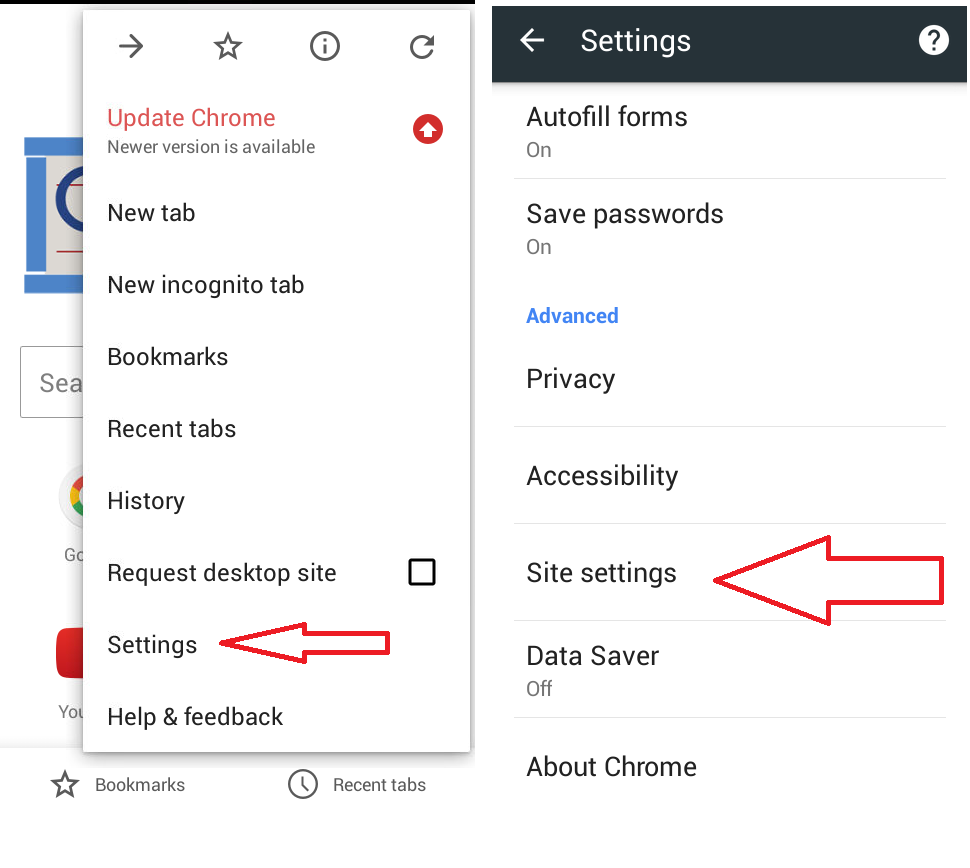In this image, we observe two distinct settings menus, likely displayed on a cell phone screen. The orientation of the menus is primarily vertical. 

On the left side of the image, the menu begins with a top bar featuring icons such as a forward arrow, a star, an info button, and a refresh button. Below this bar, the menu lists various options including "Update Chrome," "New Tab," "New Incognito Tab," "Bookmarks," "Recent Tabs," "History," "Request Desktop Site," "Settings," and "Help and Feedback."

To the right, another settings menu is visible, characterized by a black header at the top labeled "Settings" and accompanied by a back arrow. This menu includes options for "Autofill Forms," "Save Passwords," "Privacy," "Accessibility," "Site Settings," "Data Saver," and "About Chrome."

Notably, both menus feature large, red arrows pointing towards the "Settings" options, drawing attention to this specific entry in each list.